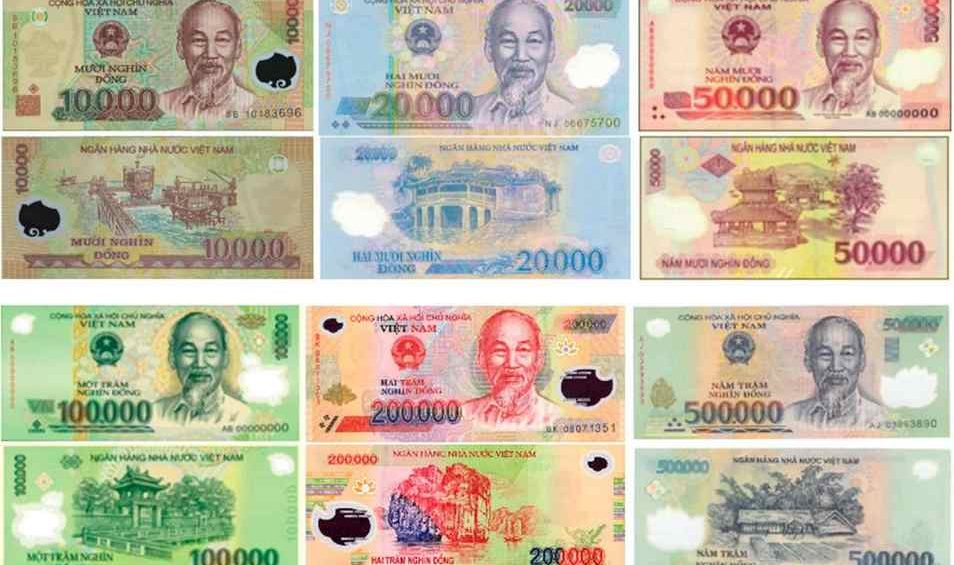This collage features 12 Vietnamese currency notes, meticulously arranged to showcase six different denominations, each displayed with both front and back views. Dominated by a range of colors—dark greens, oranges, light blues, greens, pinks, and yellows—each bill is strikingly vibrant. Common across all denominations is the portrait of a bald, Asian man with a long goatee, dressed in a white button-up shirt. The denominations prominently displayed include 10,000, 20,000, 50,000, 100,000, 200,000, and 500,000 dong. On the reverse side of the bills, intricate illustrations of buildings echo traditional Asian architecture. The meticulous design and vibrant hues make these notes not only functional but also a reflection of Vietnamese culture and artistry.